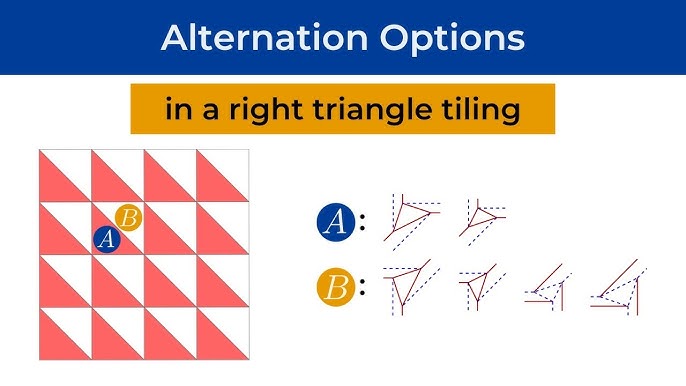The image is a detailed diagram illustrating alternation options in right triangle tiling. At the top, a wide dark blue banner with white text reads "Alternation Options." Below, an orange banner with dark blue text announces "In a Right Triangle Tiling." To the left, there is a square composed of a 4x4 grid of alternating pink and white right triangles, creating a checkerboard pattern. Below this square, two sets of circles labeled "A" and "B" are displayed: "A" is circled in blue, and "B" is circled in gold. Additionally, there are paired triangles illustrating the configuration options. Next to these, A-colon shows two triangles with lines extending from them, while B-colon shows four triangles, with two appearing partially complete via dotted and straight lines.